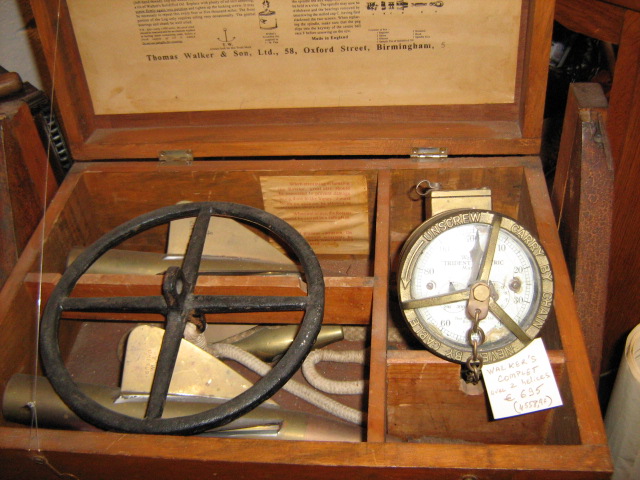"Color photograph of an antique weighing instrument housed in a handcrafted wooden box. The box, aged and with visible wear, is divided into five compartments—two large ones on the left and three smaller ones on the right. The lid of the box is open, revealing an original label on the underside that reads 'Thomas Walker and Son Limited, 58 Oxford Street, Birmingham, England.' The parchment-colored paper, yellowed with age, displays black text and an illustration resembling a hanging brass weight.

The lid is propped open, likely in a museum display, as evidenced by a piece of fishing line attached to a clasp on the box and extending upward, keeping the lid in position. On the left side of the image, partially visible, are objects that appear to be the spines of some books.

Inside the box, a circular iron frame divided into quadrants by intersecting bars is visible. A round hook adorns the center where the bars intersect, with an additional protrusion below that seems to have another hook attached. On the smaller right side compartments, a brass instrument, presumably an old-fashioned hanging scale, lies flat. This brass scale features a white face with numerous numbers and a peace sign-like arrangement of three metal pieces across its front. A dangling part and a Post-it note with some writing are attached, indicating the item is part of a curated display in what might be a museum dedicated to antique tools and instruments."